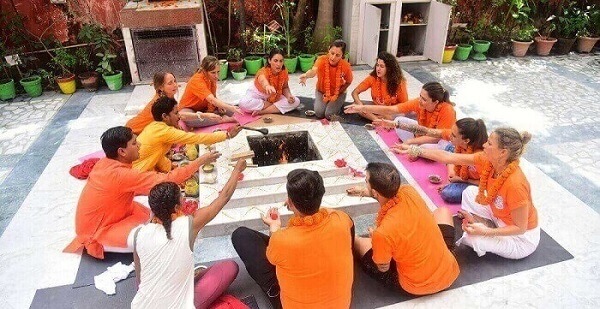This photograph captures a group of 13 people engaged in a religious ceremony at a modernistic outdoor retreat in India. They are seated cross-legged on yoga mats around a square, tiered fire pit made of marble or stone, which serves as both a hearth and communal table. Most participants are dressed in traditional saffron orange attire, symbolizing a Hindu ritual, with two exceptions: one individual in a white shirt and another in a yellowish-gold long-sleeve shirt. All participants wear orange garlands around their necks and hold objects, likely petals or food, poised over the fire, contributing to the ceremonial atmosphere. Bowls of food are arranged on the tiers of the fire pit. In the background, a wall adorned with potted plants creates a serene ambiance, framing this spiritual gathering.